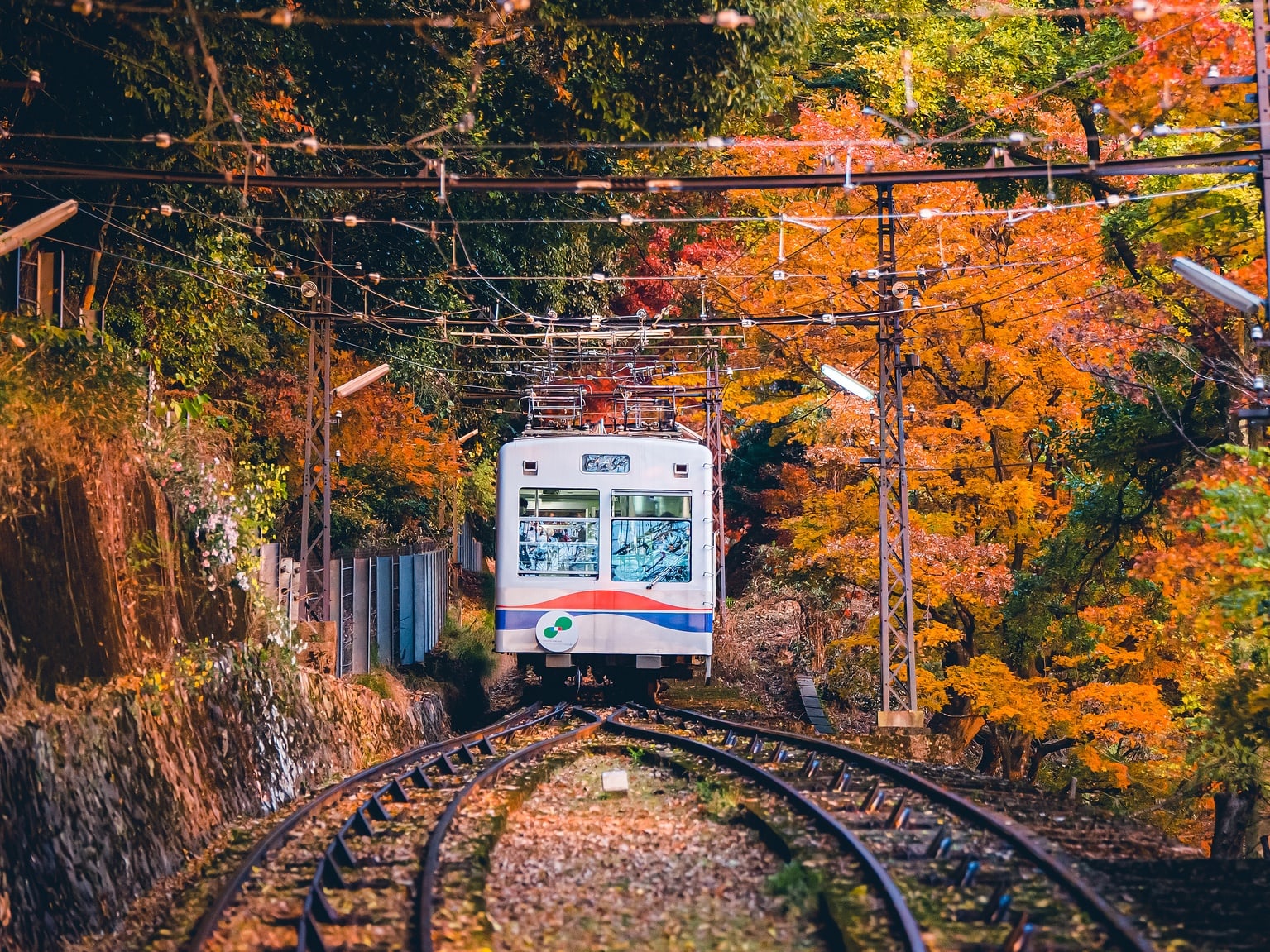In the image, we see the vivid back of a train, predominantly white with distinct red and blue accents. The train features two rear windows with small holes atop them and a smaller central window in between. The train is positioned on tracks which split into two separate lanes, curving outward. Adjacent to the tracks, which are set on a gravel path, are guiding wires suspended on small towers. The surrounding area is lush with trees bearing leaves in varying shades of green, orange, red, and yellow, suggesting a fall setting. The environment includes visible rock formations and a natural dirt wall on the left side of the tracks, enhancing the forest-like atmosphere. The right side presents more ground-level trees. It’s a sunny day, casting slight shadows on the tracks, and the scene is adorned with some trees blooming with orange and red flowers.